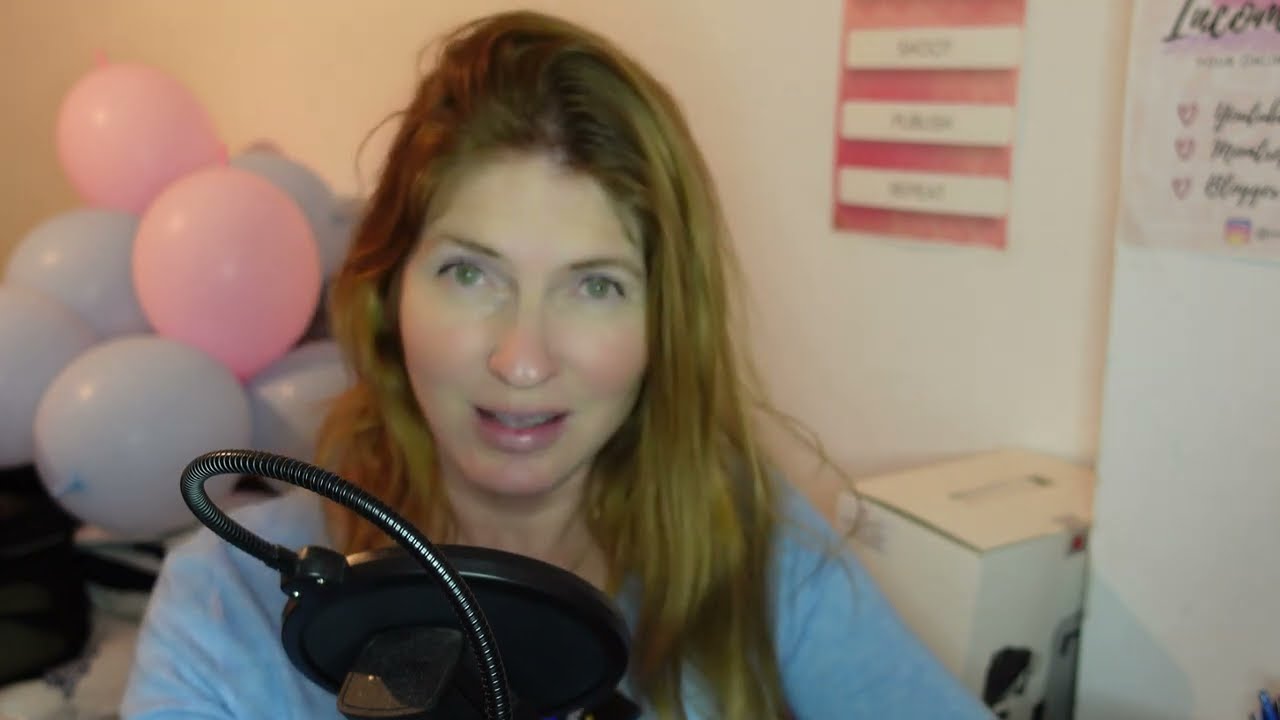The photograph features a slightly out-of-focus Caucasian woman with long, flowing light brown to blonde hair and vibrant green eyes, and thin blonde eyebrows. Her face, framed by her deep brown blonde hair, has pink cheeks and pink lips, and the tip of her nose is also slightly rosy. She appears to be in mid-conversation, with her mouth partially open, giving her an engaged and dynamic expression. The woman is dressed in a blue or a gray t-shirt and is seated or standing in a room, possibly a house or an office.

In the foreground, in sharp focus, is a black, round microphone with a pop filter and a black cord trailing from the back. Behind the woman, the room has a slightly cluttered, celebratory atmosphere with a large pile of balloons mostly in light blue and a couple in pink, positioned on the left-hand side of the image. The wall behind her is white, featuring hand-drawn signs that add a personal touch to the space, and a red and white striped object or poster adding a bit of color. There's also a white box on the floor to the right, contents unknown. The lighting in the room casts a slight yellow glow, enhancing the warm, inviting feel of the space.